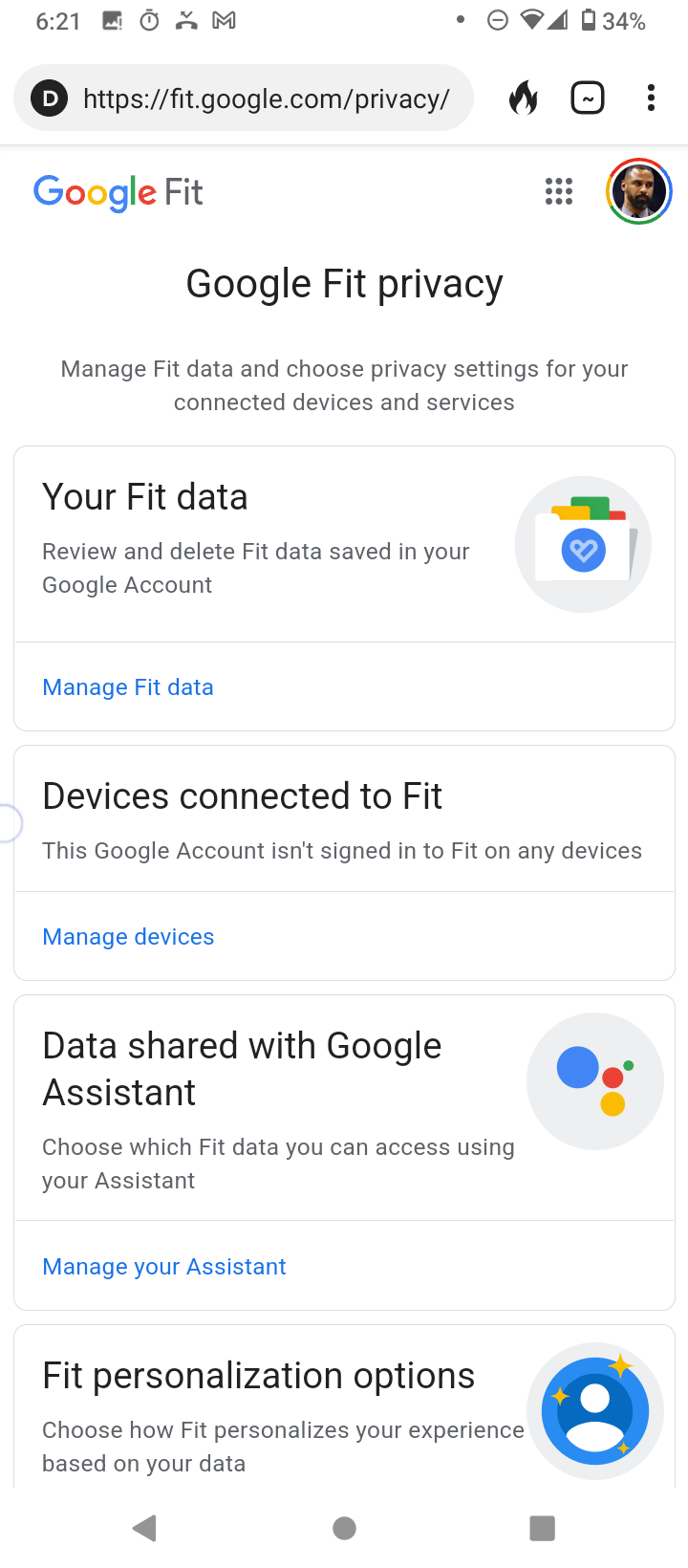This is an image depicting the settings page for Google Fit on the Google.com website, focused on user privacy. The screen showcases various tabs for adjusting privacy settings. In the upper-right corner, a profile image is displayed, and atop the screen, the time reads 6:21 with a battery level at 34%.

Centrally, the bold header reads "Google Fit Privacy" with multiple interactive tabs below it:
1. "Your Fit Data": Users can manage their fitness data by clicking the blue "Manage Fit Data" link.
2. "Devices Connected to Fit": This section lets users handle devices linked to Google Fit through the blue "Manage Devices" link.
3. "Data Shared with Google Assistant": It provides options for managing interactions with Google Assistant.
4. "Fit Personalization Options": Users can customize how their fitness data is utilized to personalize their Google Fit experience.

Below these settings, navigational options include a back button (a left-facing triangle), a home button (a dot), and a recent apps button (a square), forming a bar at the bottom of the screen. Descriptions under each header further guide users on how to navigate their privacy preferences for Google Fit.